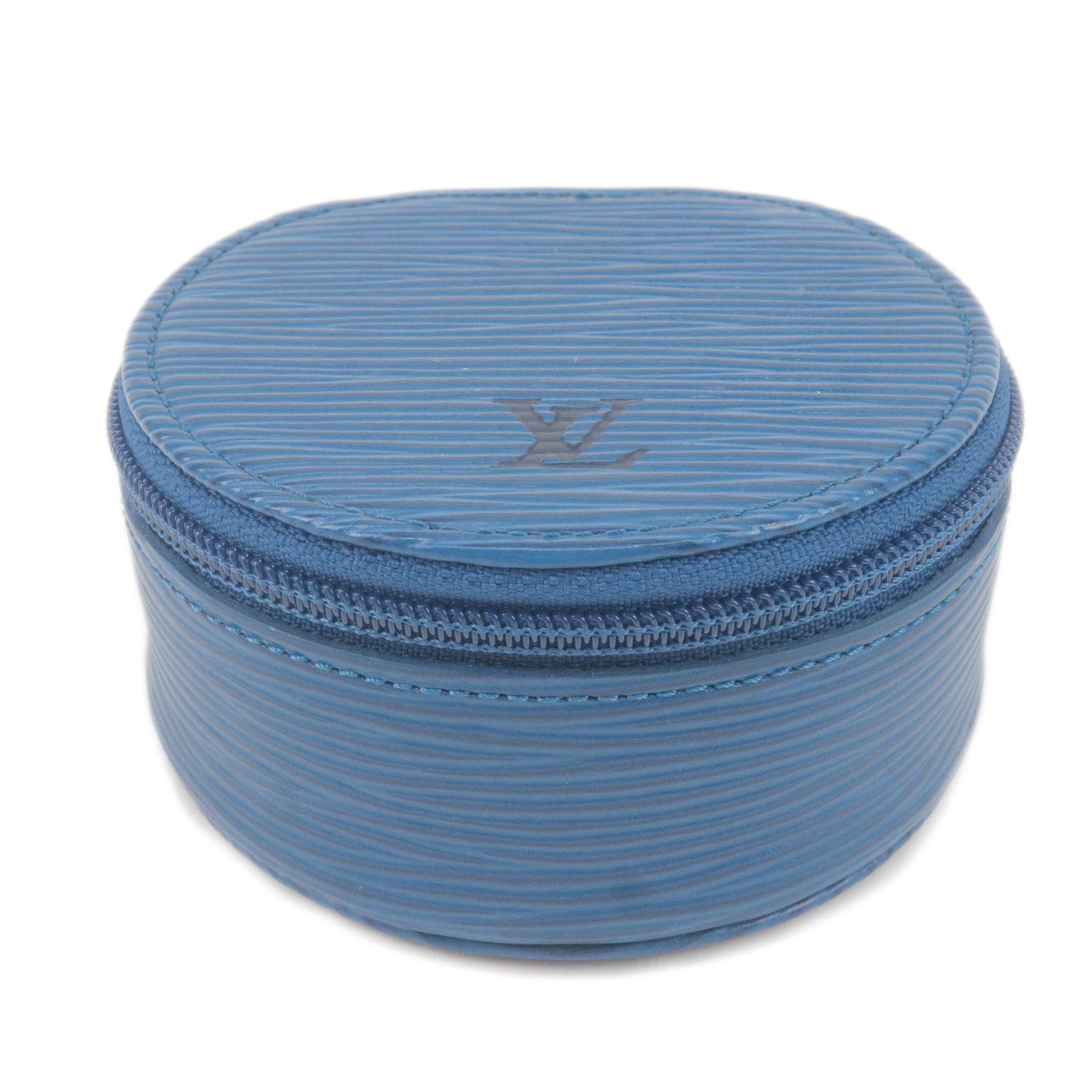The image depicts a full-color photograph of what appears to be a round, blue zippered fabric case set against a white background. The case, resembling backpack material, features a pattern of horizontal stripes in varying shades of blue and faint gray. The stripes run across both the top and bottom sections of the case. Circular stitching is visible along the edges, securing the fabric together. The case has a zipper that encircles the middle but the zipper handle is not visible. Towards the lower center of the top section, the gray initials "XL" are printed. Despite the monochrome color scheme, the details such as the zipper, stitching, and striped pattern provide a textured appearance to the case.